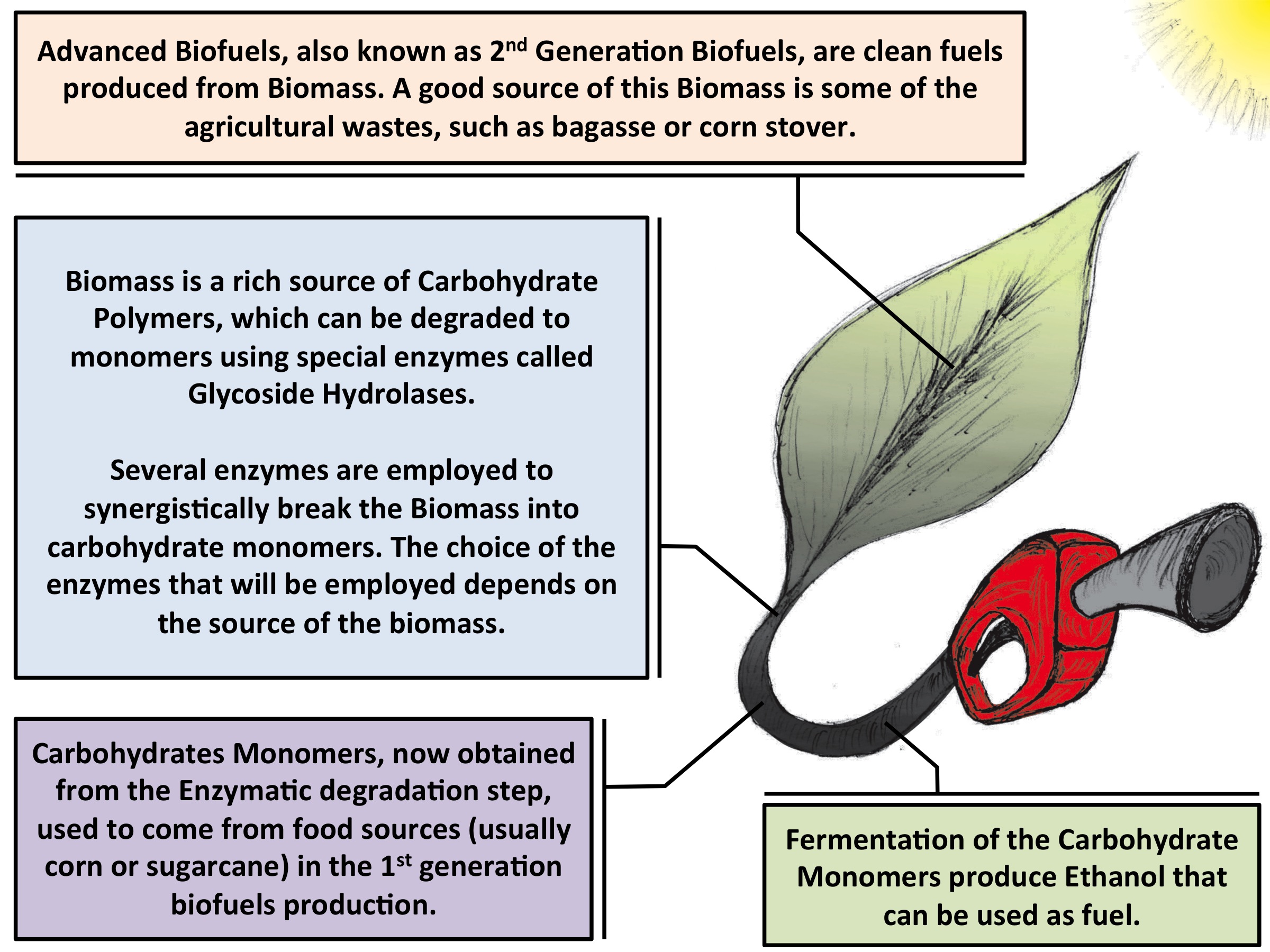This image is of an informative chart focusing on biofuels, featuring a detailed illustration of a plant leaf that seamlessly morphs into a red-handled gas dispenser, resembling those found at gas stations. The background of the image is light, with a small sun icon positioned in the top right corner, symbolizing energy. The chart is sectioned into four colored boxes, each outlining critical aspects of biofuel production. 

1. The top left box, in neutral tan, provides a definition: "Advanced Biofuels, also known as Second Generation Biofuels, are clean fuels produced from biomass. A major source of this biomass includes agricultural waste like bagasse or corn stover."

2. The light blue box underneath elaborates: "Biomass is rich in carbohydrate polymers, which can be degraded to monomers using specialized enzymes known as glycoside hydrolases. Several enzymes work together to break down the biomass, with the choice of enzyme depending on the biomass source."

3. The purple box, located at the bottom left, details the carbohydrate sources: "Carbohydrate monomers, now derived from enzymatic degradation, previously originated from food sources such as corn or sugarcane in first-generation biofuel production."

4. The bottom right box, in light green, explains the final step: "Fermentation of these carbohydrate monomers produces ethanol, which can be used as fuel."

The visual and textual elements collectively explain the process of converting agricultural waste into advanced biofuels, emphasizing the role of enzymes and the transition from food-based to biomass-based sources.